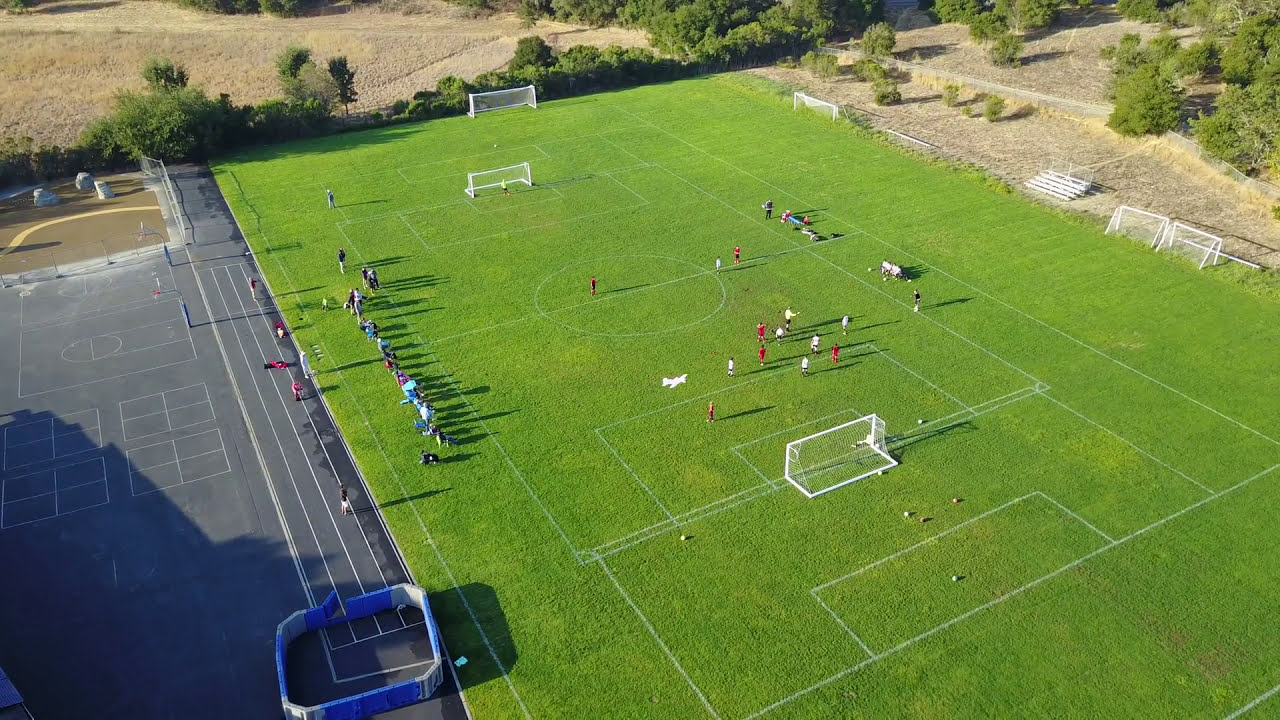This aerial shot captures a bustling recreational area centered around a large soccer field with vibrant green grass and crisp white lines. The field hosts an ongoing match featuring two teams, one dressed in red jerseys and the other in white, while a referee in a yellow shirt oversees the game. White soccer nets stand at either end of the field. On the left side of the image, spectators dressed in various shades of blue can be seen standing along the sidelines, possibly offering support or waiting their turn to play. Adjacent to the soccer field, there's a multi-use basketball court with black concrete, equipped with hoops and marked by yellow lines. Beyond the courts, towards the top of the image, stretches a large field dotted with green trees, creating a natural boundary against the tan hues of the surrounding landscape. In the top left, a parking lot marked with white lines is visible, and near the bottom of the image, there is a blue and white structure with an open door, possibly a facility or storage area. Further to the right, three more white soccer nets are seen along with some white bleachers, highlighting the area's capacity for multiple games and spectators. The overall scene epitomizes a vibrant community space, likely part of a high school or local sports complex.